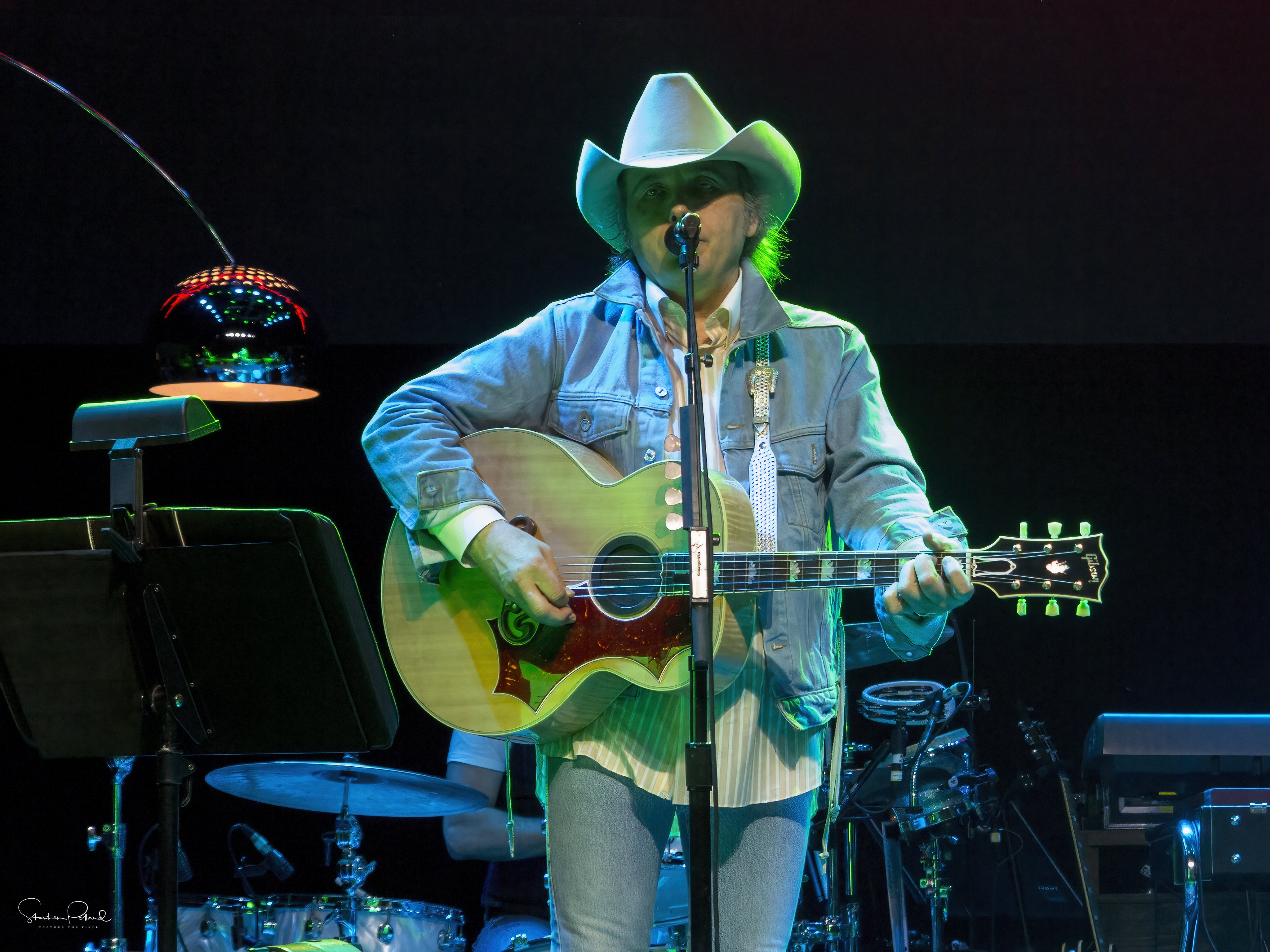A man, dressed in a light blue denim jacket with white buttons and tight blue jeans, stands on a dimly-lit stage performing. His white and gray striped button-up shirt with the collar turned down peeks out from under the jacket, while the sleeves of his jacket are slightly turned up and the wrist buttons are open. Donning a white cowboy hat, he appears to be a country or Western singer, adding to the rustic charm. In both hands, he cradles a light brown acoustic Gibson guitar, characterized by a red pick guard. The guitar looks slightly oversized, emphasizing his role as both singer and guitarist. He sings into a microphone positioned before him, attached to a black microphone stand with a flexible wire running up its side. Behind him, the barely-visible arm of a drummer and a drum set hint at the presence of a full band. There are stage lights casting a lime green hue, adding a splash of color to the scene. To his left, a music stand and an inexplicable lamp contribute to the setting. The background, consumed by solid black, accentuates the focused spotlight on this evocative musical moment.